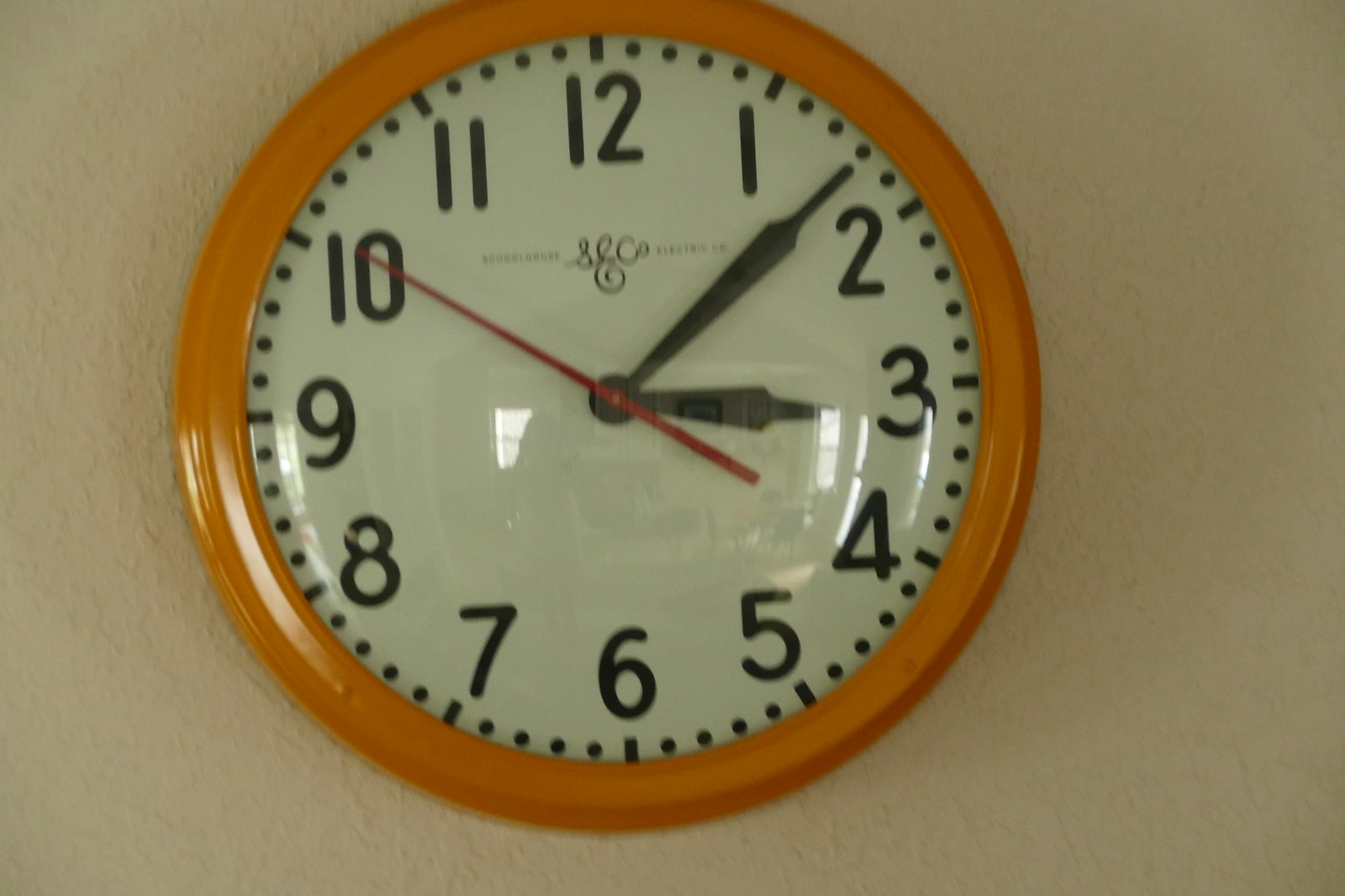The image showcases a round plastic wall clock with an orange border. The clock's face is white with black Arabic numerals clearly marking 1 through 12. Each numeral is accompanied by long ticks and four intermediate dots between each pair of numerals. The clock features four hands: a long black minute hand pointing between 1 and 2, a similarly black hour hand almost directly at 3, and a red second hand positioned just above the 10. Centered below the number 12, there's a logo and text in black, albeit slightly unclear and in cursive, possibly featuring the letters "S" and "C."